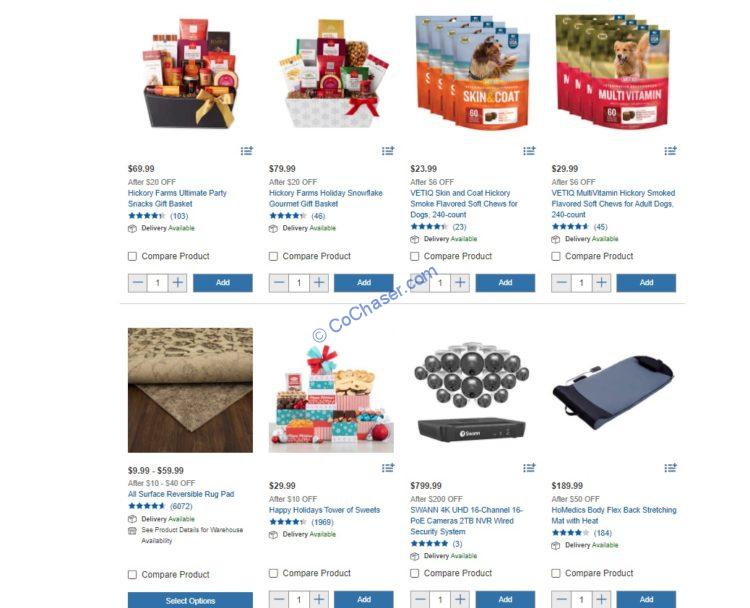The image appears to be a page from an online shopping platform showcasing a diverse range of products. At the top, there are holiday-themed gourmet gift baskets from Hickory Farms, including a holiday gourmet gift basket and a snack oak gift basket, festively arranged. The pet section features 'Skin and Coat Hickory Smoke Flavored Soft Chews for Dogs' and 'Hickory Chews for Adult Dogs', indicating an assortment of treats for canine companions. Additionally, there is a decorative rug and an array of sweets, including some delectable cakes. Under the heading "Camera," a 2TB NVR Wired Security System is displayed, possibly offering sophisticated surveillance technology. Lastly, the "Home Medics" section features a Flex Back Stretching Mat with Heat, emphasizing their health and wellness product line.